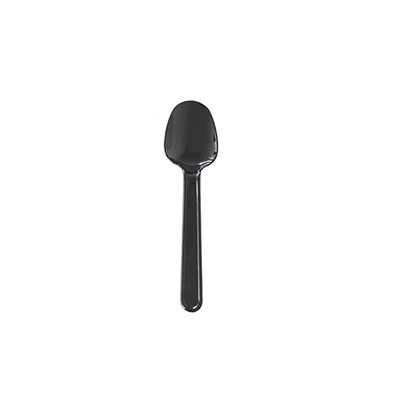The image is a professional shot of a single, black utensil set against a stark white, completely blank background. The utensil, which is centered in the frame, appears to be a dark, shiny plastic spoon or possibly a silicone spatula, creating some ambiguity. The top portion of the utensil, which could be a rounded spoon bowl or the flat working end of a spatula, is positioned at the top of the image, tapering into a consistent, wide handle that ends in a slightly rounded tip at the bottom of the image. The dark color of the utensil contrasts sharply with the white background, making it reflective and causing some white and gray highlights on the edges, especially on the right side due to the light source. This minimalist presentation suggests it could be intended for retail or website purposes, showcasing the simplicity and functionality of the kitchen tool.